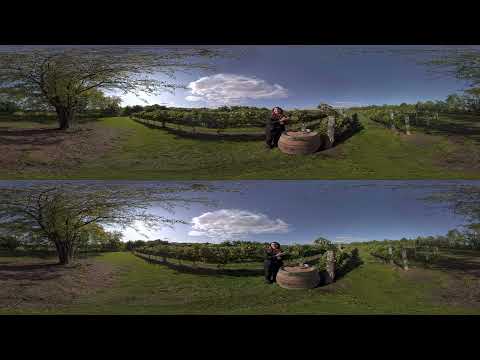The image features two identical panoramic photos stacked vertically within a single frame, bordered at the top and bottom by black bars making up about 10% of the image each. The scene captures a picturesque outdoor setting that resembles a tree farm, orchard, or possibly a vinery. At the heart of this idyllic scenery stands the figure of a woman with long brown hair, dressed in dark clothing. She faces the camera, though her face remains unseen. The woman is situated beside a wooden wine cask or barrel, placed on a vibrant green grassy field.

To the left side of the image, a large willow tree extends its cascading branches over the field, adding to the natural tranquility of the scene. The sky overhead is a lovely light blue, dotted with a few white cumulus clouds, through which sunlight filters, illuminating the entire landscape. Behind the woman lies a lush grove of greenery, contributing to the depth and richness of the setting. Although one observer speculated that the woman might be standing in front of corn or holding an animal, the overall impression remains one of serene beauty and natural splendor, captured twice in a striking horizontal orientation.